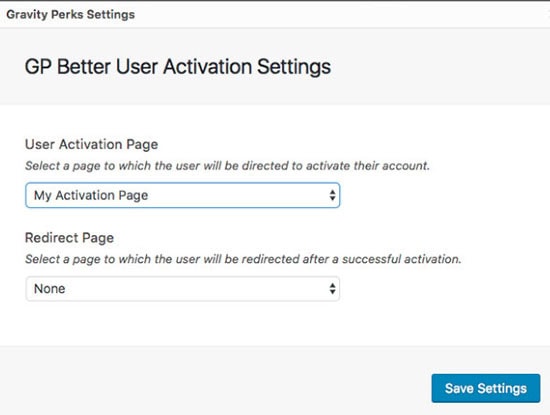**Descriptive Caption:**

The image is a cropped screenshot depicting a settings window from either a website or a software application, isolating the specific interface for detailed focus. The title at the top of the pop-up window reads "Gravity Perk Settings" in prominent black text. Directly beneath this title, a light grey rectangle displays the text "GP Better User Activation Settings."

The main section of the window has a white background and contains two scrollable input fields. The first input field, labeled "User Activation Page," allows the user to select a webpage that new users will be directed to in order to activate their account. The current selection shown is "My Activation Page." The second input field, labeled "Redirect Page," enables the choice of a webpage where users will be redirected after successfully activating their account; however, no selection has been made in this field.

At the bottom-right corner of the window, a blue "Save Settings" button is available for users to confirm and save their configuration choices.